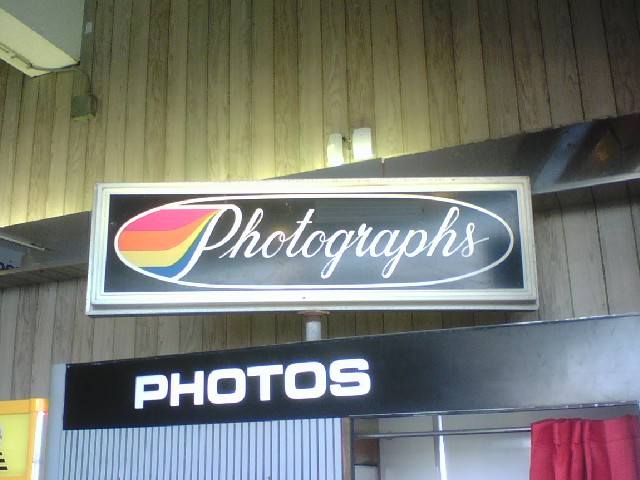The image depicts the interior of a quaint shop, focusing on the upper portion of an old-fashioned photo booth. At the top of the booth, an elongated rectangular sign with a vintage wooden frame catches the eye. The frame encloses a black background, possibly made of cardboard, featuring an elongated white oval stretching horizontally across the center. Inside this oval, the word "photographs" is elegantly scripted in cursive. Adjacent to the sign's peak, the left side is adorned with vibrant stripes in shades of pink, orange, yellow, and blue, adding a burst of color to the scene.